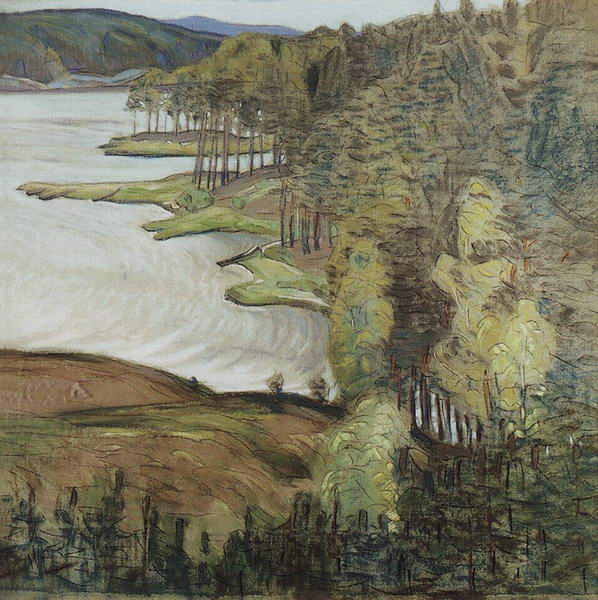The painting depicts a serene, impressionist-style landscape reminiscent of works by Van Gogh or Monet. Dominated by muted earth tones, it features an array of browns, greens, and soft yellows. A large body of water lies to the left, its surface a neutral white rather than blue, capturing the subtle play of light. The scene transitions to a forested area on the right, with darker tree trunks framed against lighter foliage as the perspective recedes. The background is filled with rolling mountains or large hills, adding depth to the terrain. The painting employs thick, textured paint strokes that suggest a tangible roughness, emphasizing the flow of the water and the ruggedness of the terrain. There are no human figures present; the focus is entirely on the natural beauty of the landscape, with particular attention to the interplay of colors and textures. The sky is minimally visible, further concentrating the viewer's attention on the detailed depiction of nature's elements.